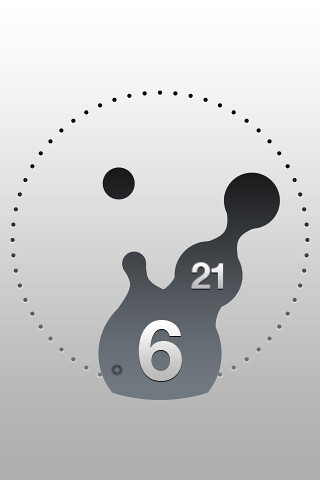The image features an abstract digital clock set against a gray background. Central to the composition is a circle formed by small black dots, approximately an inch and a half in diameter. Inside this circle, near the upper left sector, sits a significant dot about the size of a pencil's diameter, alluding to a celestial body like the sun or moon. Adjacent to this dot, towards the right, lies a larger, irregular black shape resembling two connected bottles or a tipped-over bowling pin, creating an impression of a pooling black paint. Embedded within this black mass are the numbers "21" at the top and a much larger "6" at the bottom, both in silver or white, suggesting the time 6:21 in an abstract manner.